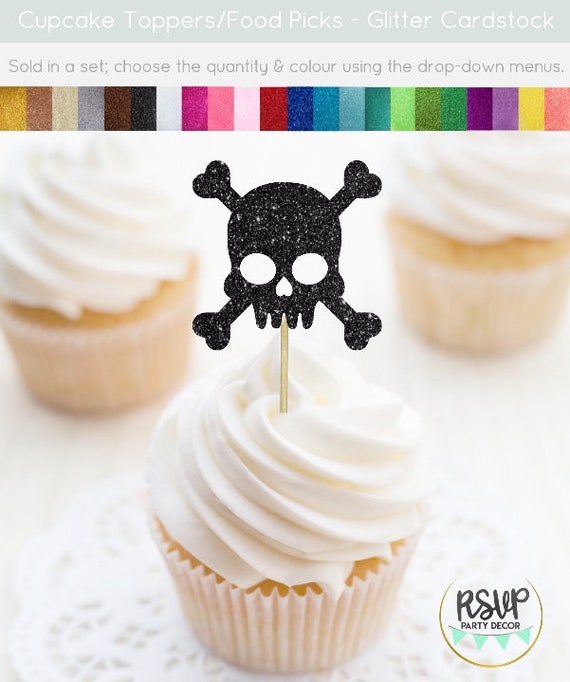The image appears to be a photographic advertisement, set indoors, showcasing various cupcake toppers and food picks available from Glitter Cardstock. At the top of the image, white text reads: "Cupcake Toppers/Food Picks - Glitter Cardstock. Sold in a set; choose the quantity & color using the drop-down menus." Below this text, a series of horizontal bands displays a wide range of colors, including gold, silver, brown, black, white, pink, light pink, burgundy, blue, dark green, light blue, greens, purples, yellow, and orange, indicating the available color options for the toppers.

The central focus of the image is a cluster of three cupcakes arranged in a triangular formation, with the front cupcake prominently displaying a black skull and crossbones topper. This topper is detailed with an upside-down heart for the nose. The cupcake itself is adorned with white, peaked vanilla frosting and encased in a white paper wrapper. Beneath the front cupcake, there are small doilies for decorative effect. The two cupcakes in the background resemble the front one but do not feature any toppers.

In the bottom right corner of the image, a graphic features blue triangular banners with the text "RSVP party decor," further establishing the branding of the product. The overall image is clear, in full color, and illuminated with bright, natural light, enhancing the visibility and appeal of the cupcake toppers.